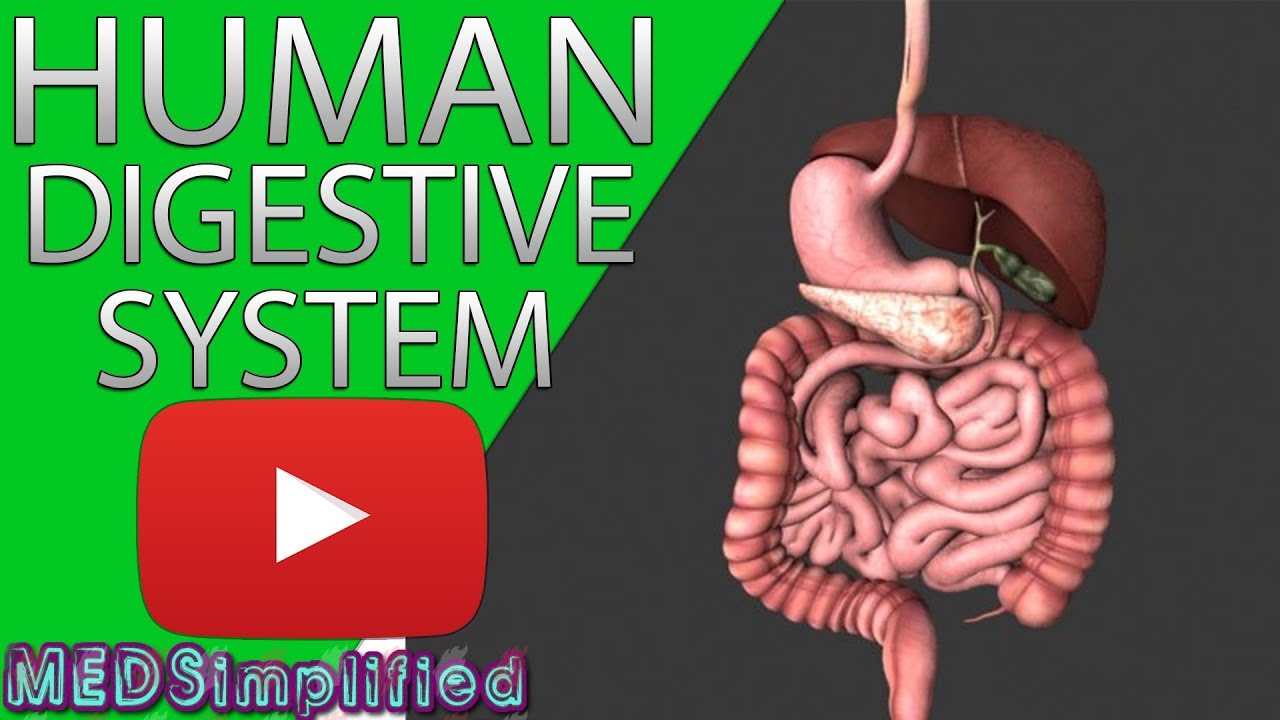The image is a detailed, graphic diagram of the human digestive system, depicted in pink and brown tones, covering the entire right side of the rectangular frame from top to bottom. The background is split, with a green left half and a charcoal gray right half. On the upper left corner, bold white text reads "Human Digestive System," beneath which is a prominent red YouTube play button featuring a white triangle. Below this play button are the words "Med Simplified" rendered in blue and purple letters. Various organs, including the stomach, intestines, and perhaps the kidneys, are illustrated against a darker backdrop, creating a clear and informative visual of the digestive system layout.